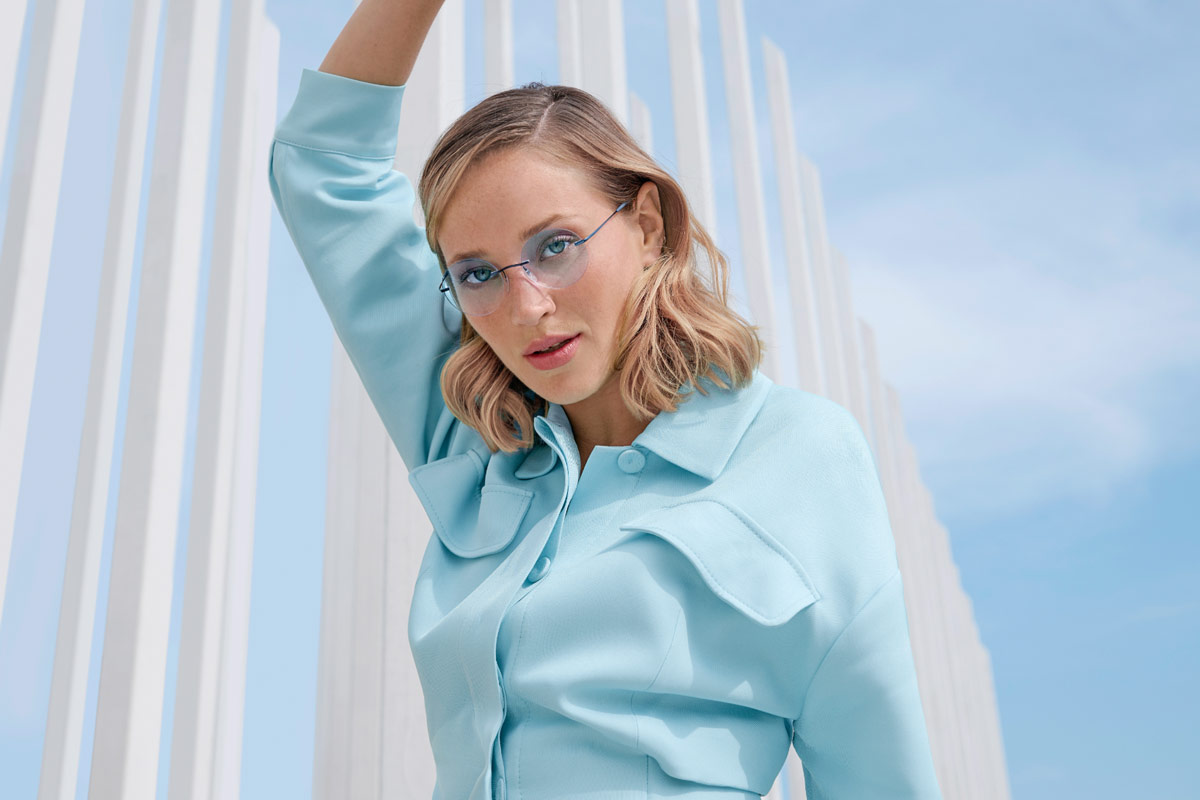In this detailed close-up image, we see a woman with blonde, wavy hair that has darker roots, styled into a deep side part. She wears rimless, blue-tinted glasses that highlight her blue eyes and accentuate a slightly open mouth with light pink lips. She is dressed in a light blue button-up dress shirt, the top button of which is undone, which has a pocket on the right side and features three-quarter sleeves. Her right arm is raised and bent above her head, though her hand is not visible in the frame. The background consists of a pale blue sky adorned with wispy white clouds and several tall, thin, white vertical pillars or sculptures varying in height, lending an artistic and modern flair. The overall impression is one of sophistication and subtle allure, as she gazes directly into the camera with an unreadable, slightly seductive expression.